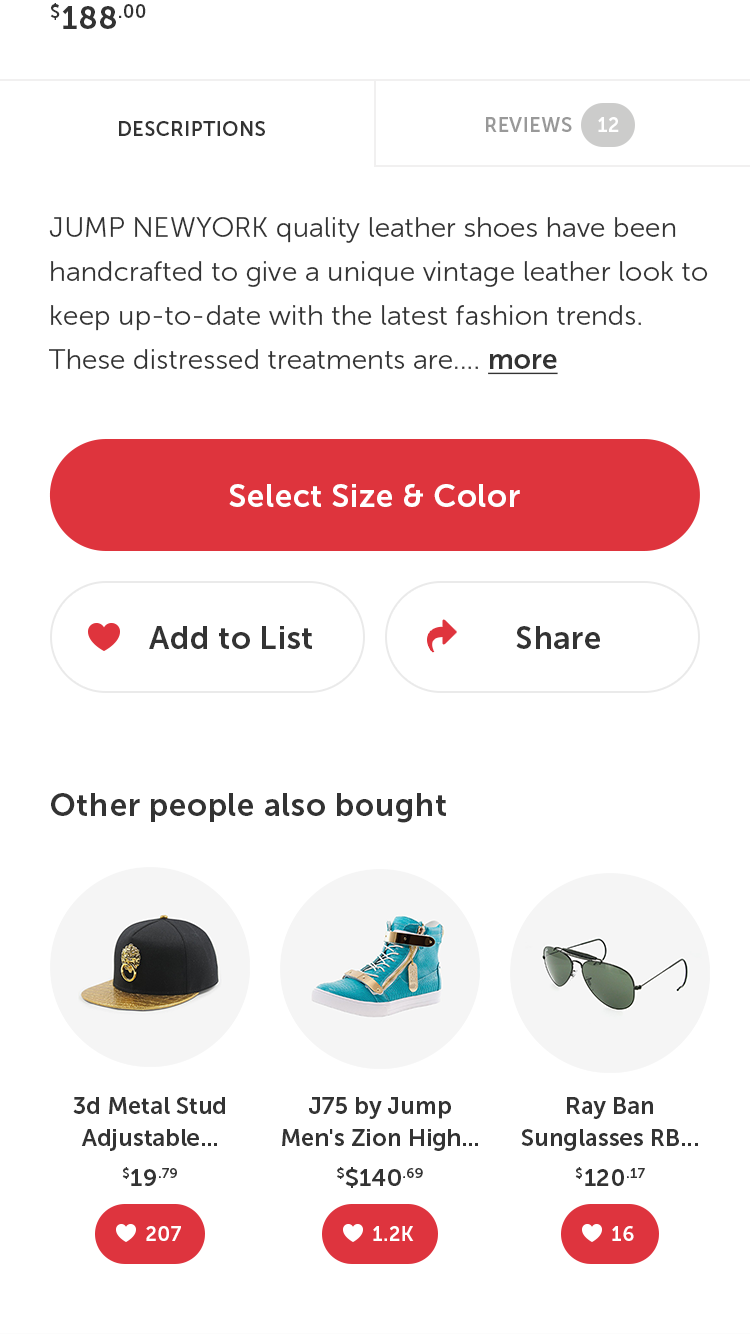The image depicts a product page from a sleek, modern e-commerce website showcasing a pair of "Jump New York" quality leather shoes, priced at $188. The image is partially cut off, but details about the shoes are visible, including a description highlighting their handcrafted construction and unique vintage leather look. The page features 12 reviews, accessible by clicking a tab, and offers options to select size and color, add the product to a list, or share it with others. Below the main product section, there's a "Customers Also Bought" section, displaying complementary items: an adjustable 3D metal stud cap for $19.79 with 207 likes, another pair of shoes for $140, and Ray-Ban sunglasses priced at $120 with 16 likes. The website's design is characterized by sleek, rounded buttons and a less cluttered interface compared to platforms like Amazon.